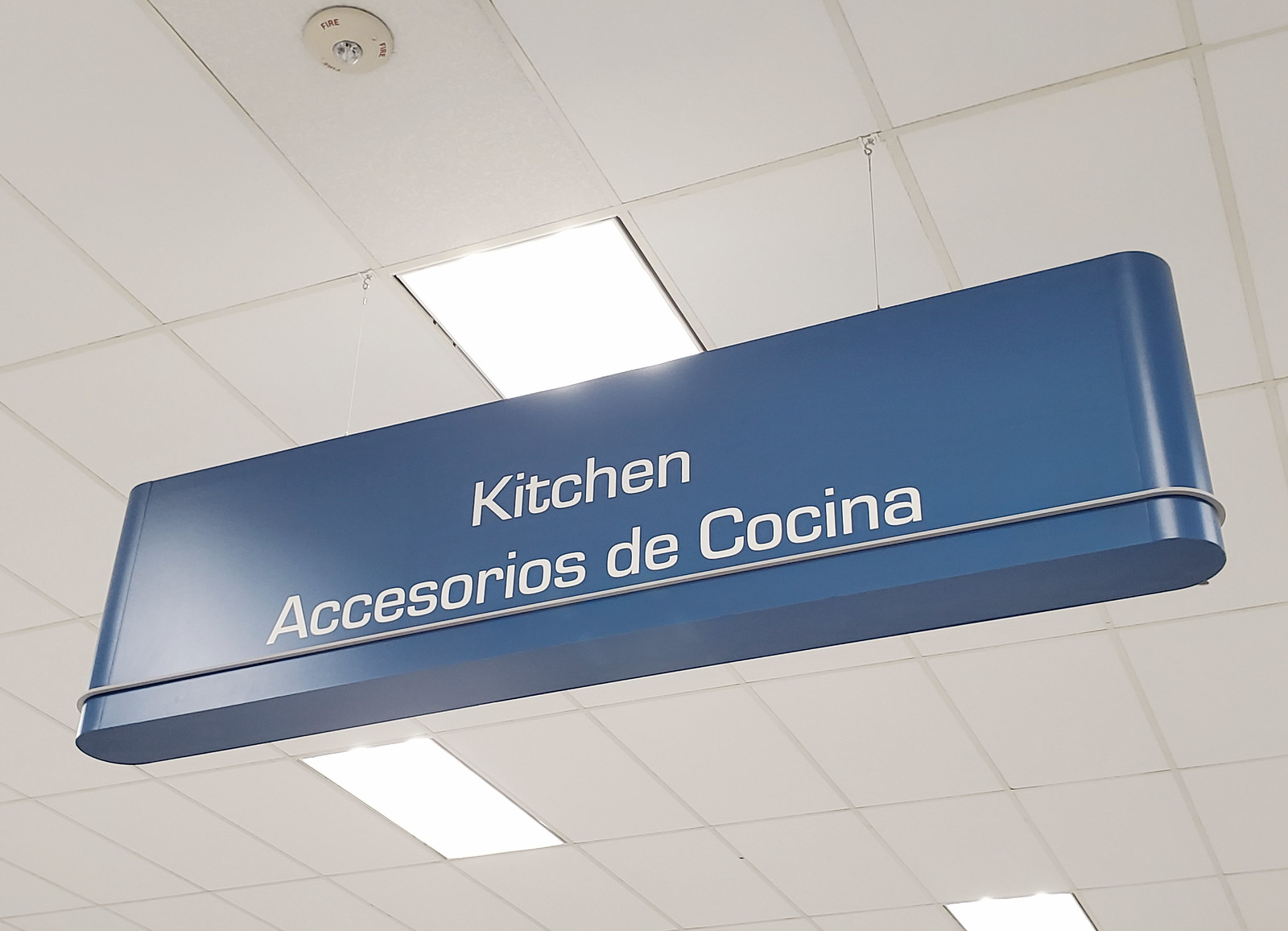The image depicts a scene inside a department store, specifically focusing on a hanging sign that designates sections within the store. The sign is suspended from the ceiling by two wires and is a medium blue color. It reads "Kitchen Accessories" along with the Spanish translation "Accessorios de Cocina." The ceiling appears to be a dated drop ceiling, featuring three fluorescent light fixtures that provide illumination. Additionally, a fire alarm is visible affixed to the ceiling. The overall ambiance suggests an older store layout designed to guide customers to various departments.